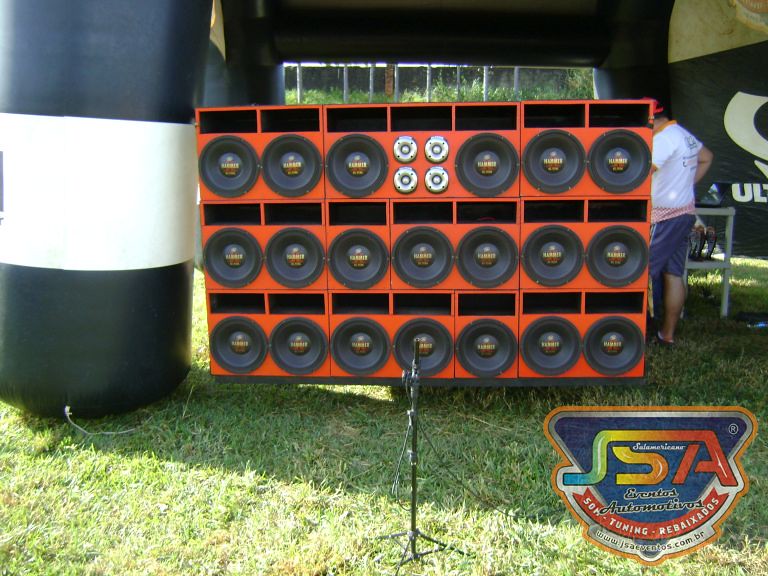The photograph captures an outdoor display set up in a large grassy field, housed within an inflatable tent with distinctive tubular black and white striped pillars. At the center of the image is a striking array of orange speaker boxes organized in a cabinet. This cabinet features three rows of seven subwoofers each, creating a grid of black, large cone-type speakers. However, the top middle row diverges from the pattern with four smaller, silver circles that may serve a different audio function like tweeters. In the forefront, you can see the base of a stand and noticeable details of a gentleman in a white shirt, blue knee-length shorts, tennis shoes, and a red ball cap, engrossed in looking over a table. Additionally, the cabinet includes an embossed logo situated in the bottom right-hand corner with text that appears to read "JSA Automotives Tuning." A website URL is present, though it is too blurry to discern. The inflatable tent's side also features a partially visible white logo on a black backdrop, associated with automotive and audio events, though it is not fully readable due to cropping.